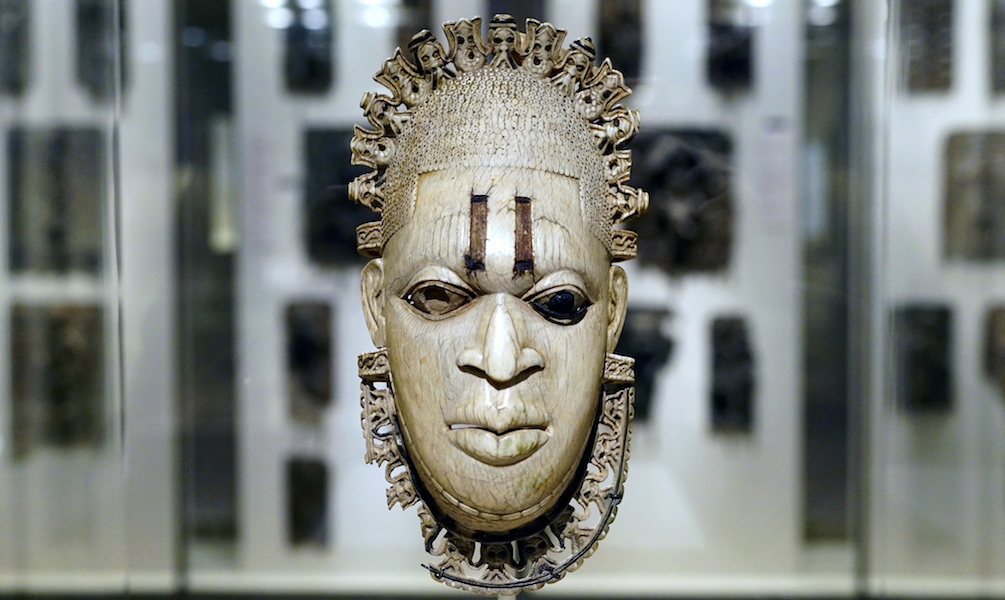This professional photograph captures a remarkable, intricately detailed mask displayed in a museum exhibit case. The mask, which is light brown in color and appears to be made of wood, depicts the face of a man with dark black eyes, a wide nose, and full lips, suggesting African origin and possibly signifying royalty or a ritualistic purpose. Notably, the mask is adorned with a detailed headdress featuring mini faces encircling the top, and around the neck, it has additional smaller faces incorporated into its design. A broken necklace is also part of the mask, emphasizing the craftsmanship. The mask is encased in a glass box, placed against a backdrop of other blurred artifacts that subtly highlight its significance and the professional composition of the photograph.